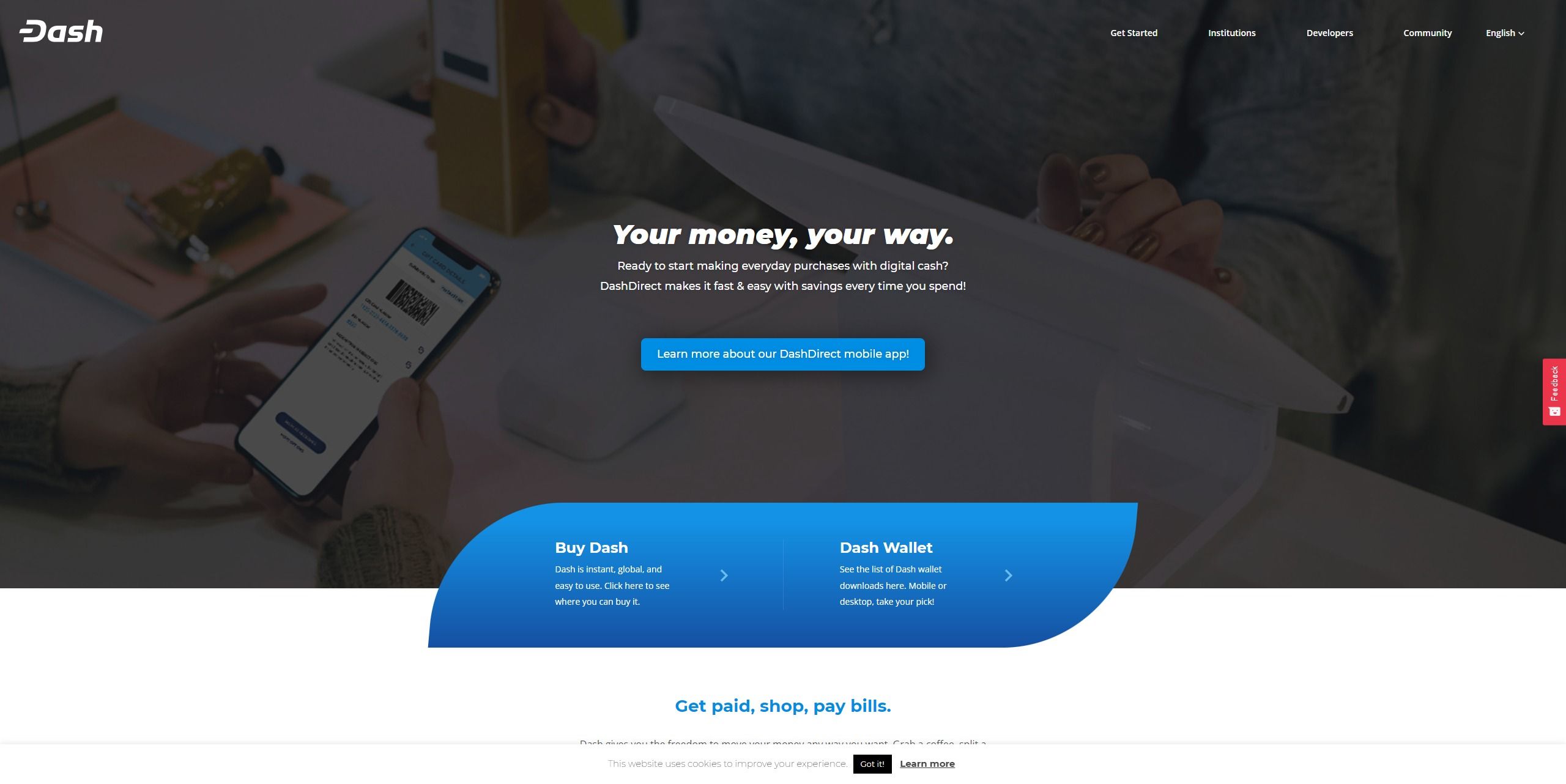This image, sourced from a website, is designed with a layered, slightly hazy overlay. The composition is rich in both visual and textual details, creating a comprehensive and engaging user interface.

**Top Section:** 
- In the top left corner, the headline "DA_SH" uses a unique typographic design where the 'D' lacks a connecting line on the left side, seamlessly integrating the dash within the word. 
- On the top right, there is an intuitive navigation menu starting with a dropdown tab labeled "English," followed by links to "Community," "Developers," "Institutions," and "Get Started."

**Center Section:**
- Centrally positioned, in bold white text, the primary tagline reads, "Your money, your way."
- Beneath it, in smaller white text, the subheading questions, "Ready to start making everyday purchases with digital cash?"
- This is followed by the text, "Dash Direct makes it fast and easy, with savings every time you spend!" accompanied by an exclamation mark to emphasize enthusiasm and ease of use.

**Call-to-Actions:**
- Directly below these texts, there is a blue rectangular button with white text inviting users to "Learn more about our Dash Direct mobile app."
- To the left, a rounded rectangle with bolded white text prompts users to "Buy Dash," supplemented with three smaller lines of explanatory text.
- To the right, another similarly styled section offers information on "Dash Wallet" with accompanying details.

**Interactive Elements:**
- A distinctive red feedback tab vertically aligned on the far right margin, with the word "Feedback" inscribed in white, offers an interactive engagement point for users' input.

**Visual Imagery:**
- The central image features a person's left hand interacting with a laptop, suggesting active use or setup, while their right hand holds an unidentified object, further indicating multitasking on a white desk.
- In the bottom left corner of the visual, two additional hands are prominently displayed holding a smartphone. The overlaid text in blue reads, "Get paid, shop, pay bills," followed by two more lines of detailed information.

This image captures a dynamic and informative glimpse into the usability and features of Dash's services, blending practical information with a user-friendly and aesthetically pleasing design.